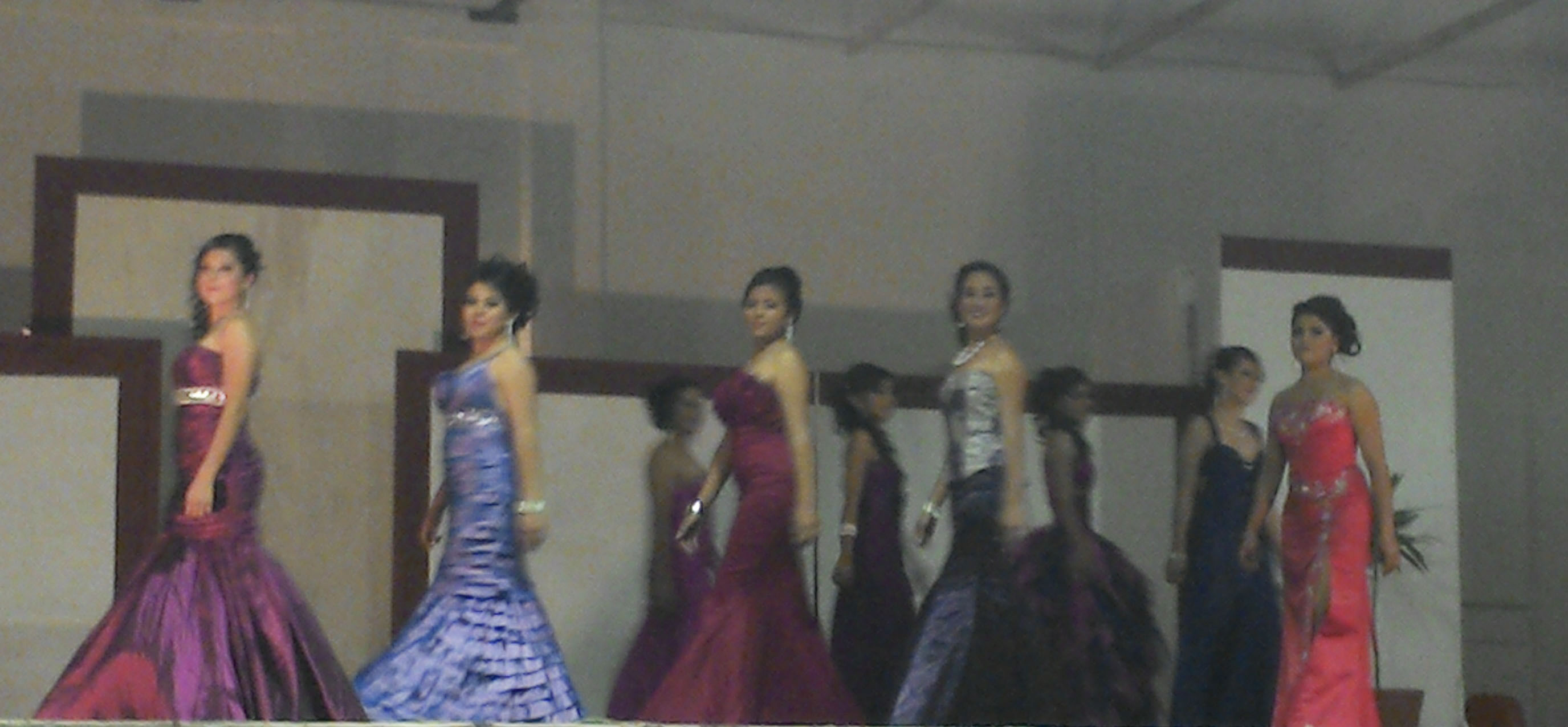In this image, a group of nine women are captured walking in a single file line, wearing elaborate and colorful gowns. The setting appears to be indoors, possibly during a daytime event like a beauty pageant or prom, given the fanciness of their dresses. The women are centrally positioned in the image, facing the camera while walking towards the left side. 

The backdrop consists of a plain white wall adorned with blank posters and brown rectangular borders or shapes providing a geometric pattern. The ceiling is notably high, estimated to be around 10 to 12 feet. The scene is well-lit, though slightly dim and somewhat blurry. 

The women's attire is vibrant and varied: the first person wears a sleeveless, strapless purple dress with a white sparkling waistband, and a flared bottom. Another flaunts a bluish gown with a similarly expansive lower half. Others are seen in dresses of pink with silver sparkles, blue with a silver top, and additional purple gowns. Notably, all the dresses share a characteristic feature of flaring out at the bottom, adding to the elegant and regal vibe of the image.